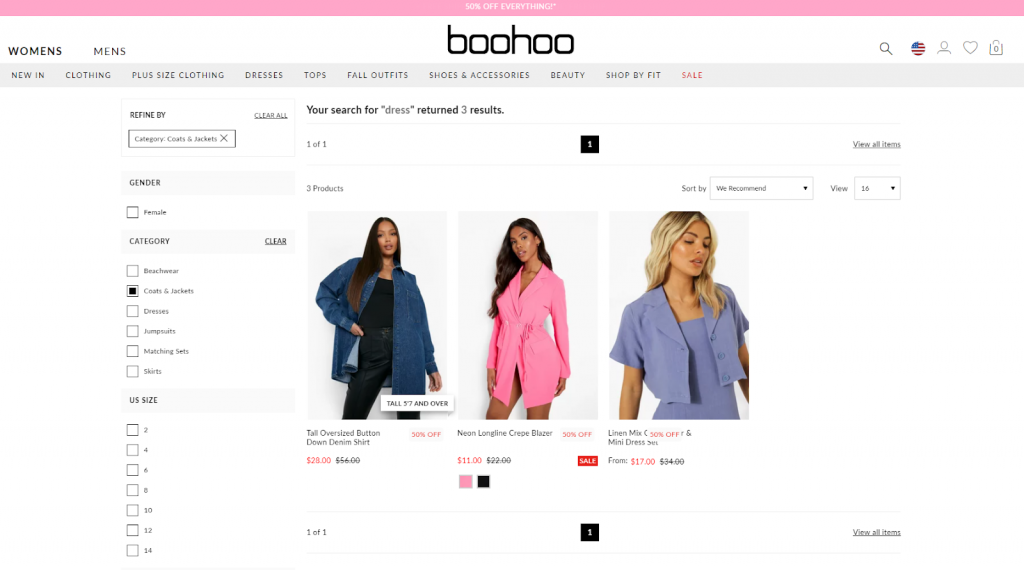The screenshot depicts a web page from Boohoo.com.

In the upper right-hand corner, the navigation options include 'Women's' and 'Men's', with 'Women's' currently highlighted in bold. There are also icons for search, country selection, user profile, wish list, and shopping cart.

Beneath the main navigation, additional categories are listed: New In, Clothing, Plus Size Clothing, Dresses, Tops, Fall Outfits, Shoes & Accessories, Beauty, Shop by Fit, and Sale. The 'Coats & Jackets' category is highlighted, indicating a refined search option. Other categories listed on the left-hand side include Beachwear, Dresses, Jumpsuits, Matching Sets, and Skirts. US sizes available are 2, 4, 6, 8, 10, 12, and 14, but none are selected.

The page features images of three Black women modeling different outfits. One wears a tall, oversized button-down denim shirt, offered at a sale price of $28, down from $60 (50% off). Another model sports a neon lounging crepe blazer in pink, priced at $11 on sale (normally $22), available in both pink and black. The third woman showcases a linen mixed seed mini dress, a blue mini dress priced at $17. All models appear on Page 1 of 1, with an option to view all items at the bottom right-hand side of the page.

Two of the women have black hair, while the third has hair with blonde tips.